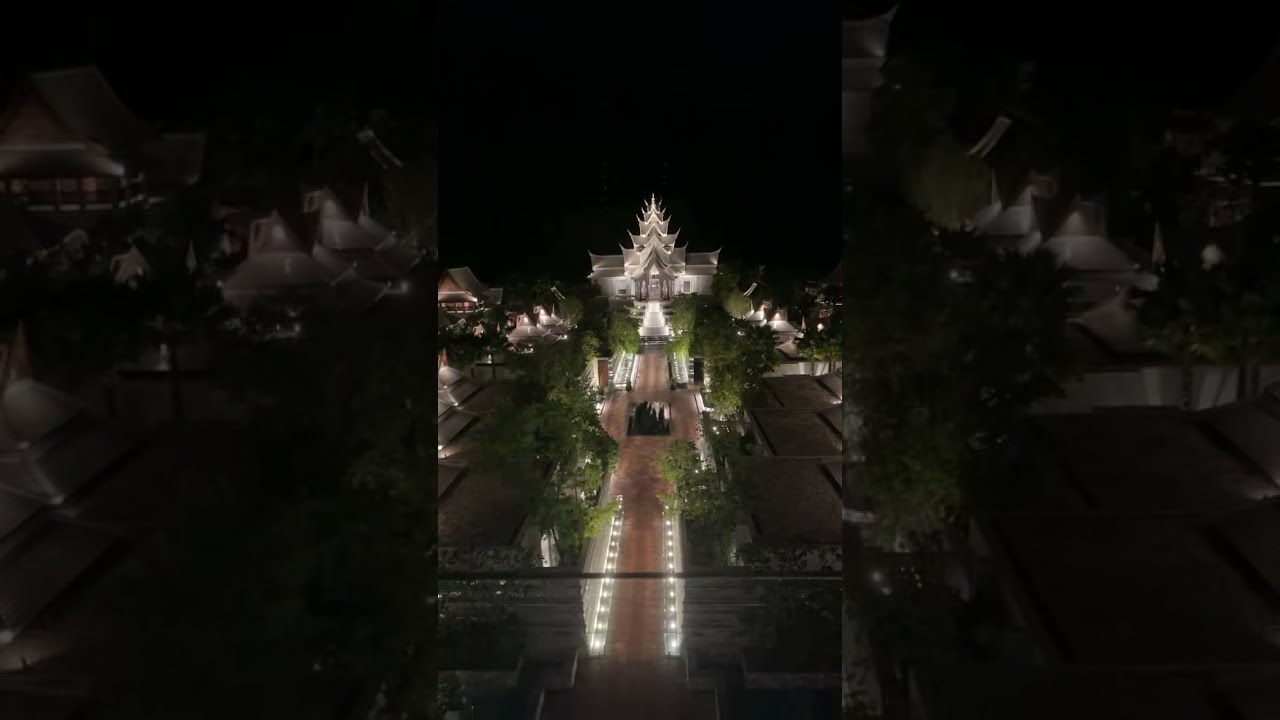The image is a very wide rectangular photograph taken at nighttime, with a completely black background. In the center, there is a tall rectangular aerial view of a grand white building, which resembles a castle, mansion, or ornate temple. This central building is highly detailed, with a middle section that is very decorated and tapers off as it rises to a pointed top. The building is illuminated by numerous white lights, making it stand out against the dark sky.

Surrounding the central image are two slightly wider, tall rectangular images that are close-up shots of the middle photograph but are shaded much darker. These images emphasize the intricate details of the central structure and its surroundings.

Stretching from the base of the central building all the way down to the bottom of the photograph is a lit pathway. This walkway is bordered by white lights on both sides and is flanked by greenery and trees. In the foreground, there is a glass railing that suggests the photograph may have been taken from a balcony. The entire setup gives the impression of a meticulous nighttime scene, possibly taken from an aerial perspective or as a still shot from a travel video, capturing the majestic beauty of the illuminated structure and its serene surroundings.